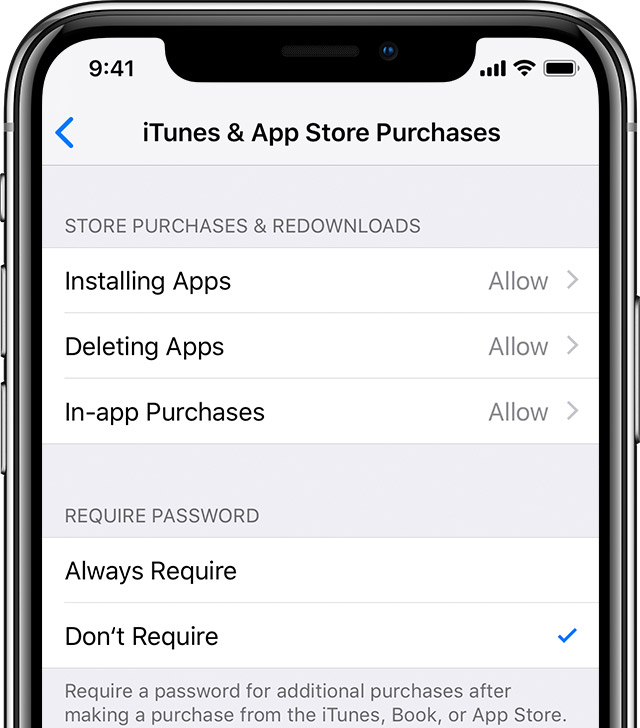The close-up image captures the top half of an iPhone screen, possibly intended as a stock or instructional photo. The screen prominently displays the "iTunes & App Store Purchases" settings page. The iPhone's status bar indicates a full battery, Wi-Fi connection, and full cellular coverage, with the current time being 9:41 AM. A blue arrow on the screen suggests a navigation option to go back to the settings menu.

Under the headline "iTunes & App Store Purchases," in gray text, it lists several options: "Store Purchases and Redownloads," "Installing Apps: Allow," "Deleting Apps: Allow," and "In-App Purchases: Allow." At the very bottom, against a white background, the text "Require Password" appears with two options: "Always Require" and "Don't Require," the latter marked with a blue checkmark. Further down in smaller gray text, it specifies, "Require a password for additional purchases after making a purchase from the iTunes, Book, or App Store."

The iPhone itself is a silver-gray model, and the backdrop is a clean, white surface, suggesting the image was professionally taken. There are no people or other elements visible in the photograph.